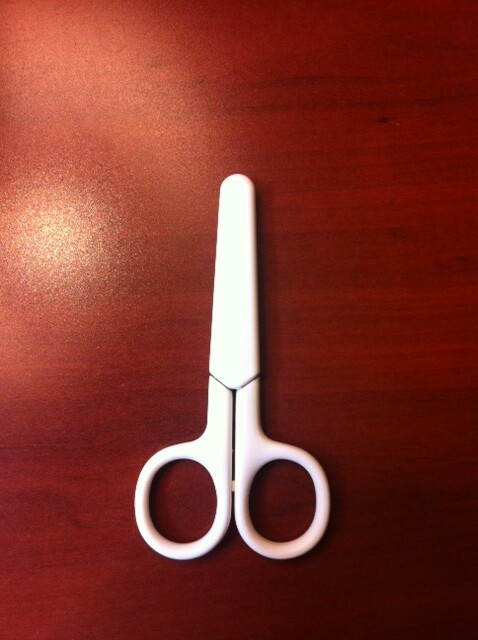The image depicts a pair of small, white safety scissors designed for kids resting on a cherry wood desk. The scissors are centrally positioned with their handles featuring small finger holes, and they remain closed under a protective white blade cover, giving them a pristine, new appearance without any scuffs. The cherry wood desk serves as a smooth, flat background, characterized by its rich red-brown mahogany hue, natural wood grain patterns, and horizontal lines, which add depth to the surface. A bright light reflection is visible at the top left corner of the desk, enhancing the texture and color of the wooden surface. The photograph is taken from a top-down perspective, capturing the neat and secure positioning of the scissors on the desk.